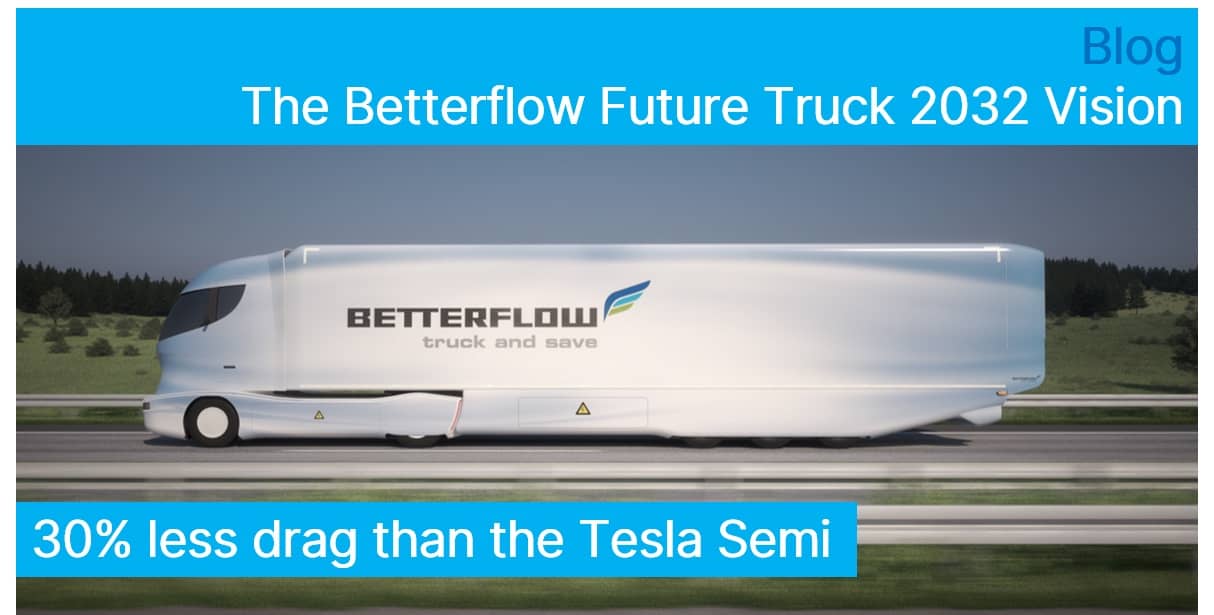The image, intended for an advertisement, features a futuristic and aerodynamic white semi-truck labeled "Better Flow Truck and Save" on its side. The truck, which appears to be a 3D rendering, is sleek and modern with a curved, helmet-like front and covered wheels, emphasizing its advanced design. It is driving down a freeway with trees and grass visible in the background, creating a picturesque countryside setting. The advertisement prominently displays a large blue banner at the top that reads "Blog: The Better Flow Future Truck 2032 Vision." A smaller blue banner at the bottom left-hand corner highlights the truck's superior performance with the claim "30% less drag than the Tesla Semi," suggesting its more efficient aerodynamic capabilities. The overall layout is longer horizontally than it is tall, giving the image a widescreen appearance.